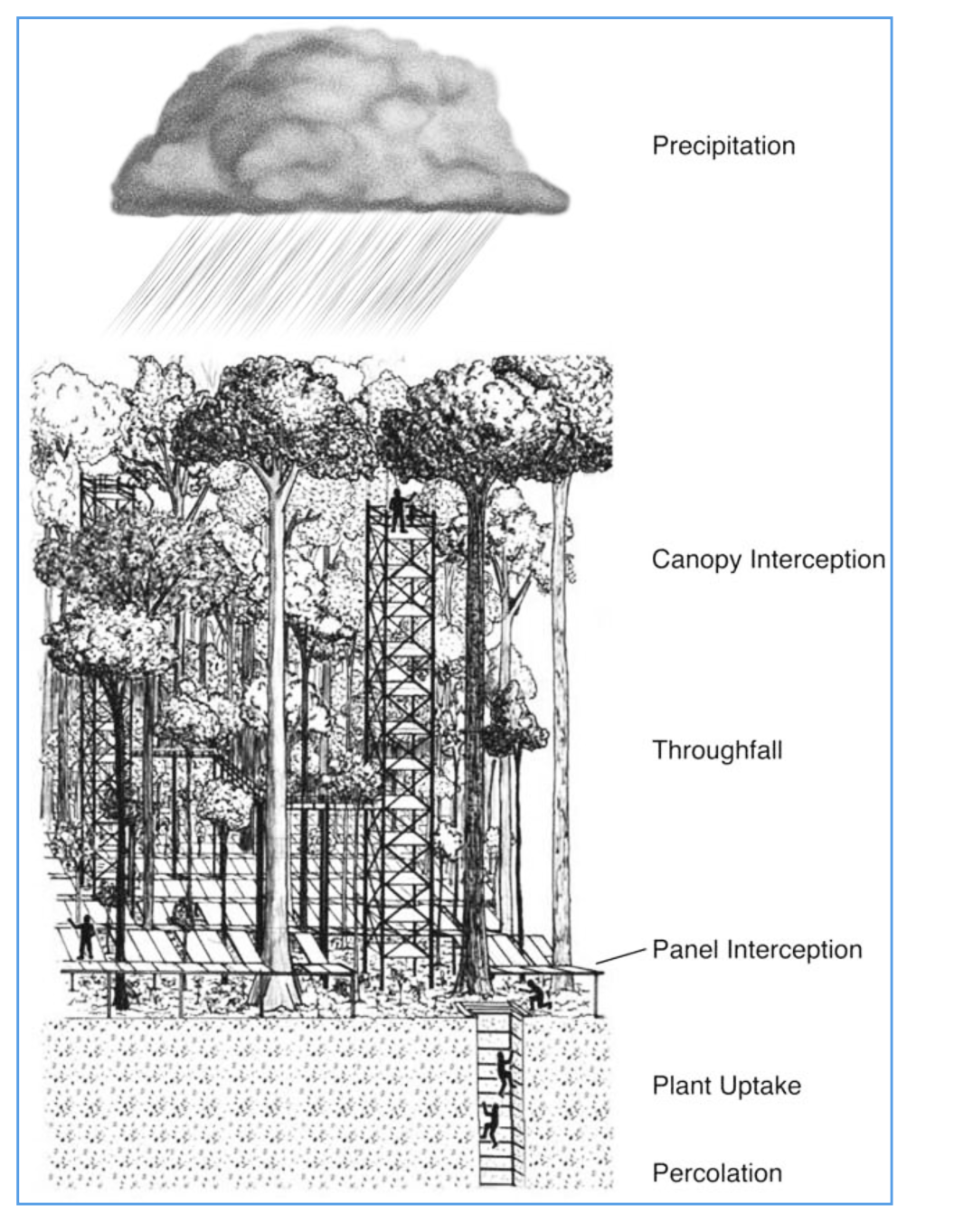This black and white diagram, surrounded by a thin blue rectangular border, illustrates the various layers and processes within a forest canopy ecosystem. At the top left, a thick gray storm cloud releases dark streaks of rain, annotated as “precipitation,” which falls slightly angled to the left onto the canopy of tall trees below. These trees, with massive trunks and dense, round leaves, form a continuous canopy intercepted by rain, labeled as "canopy interception."

Amongst the trees, a complex scaffolding structure reaches into the canopy with platforms at various levels allowing people to work. These platforms, indicated as “panel interception,” are positioned above the ground, with tree trunks extending through holes in the structure. Below this setup, the soil is depicted, with a specific section showing a tunnel on the right side where small black figures are seen climbing in or out.

The diagram labels several layers of interaction: starting from the top with “precipitation,” moving down to "canopy interception," then “throughfall” where rainwater passes the canopy. The platform level is marked as “panel interception,” proceeding to the ground level with “plant uptake,” and culminating in “percolation” within the soil. The diagram provides a clear depiction of the rainwater’s journey through the forest ecosystem and the human interaction within this environment.